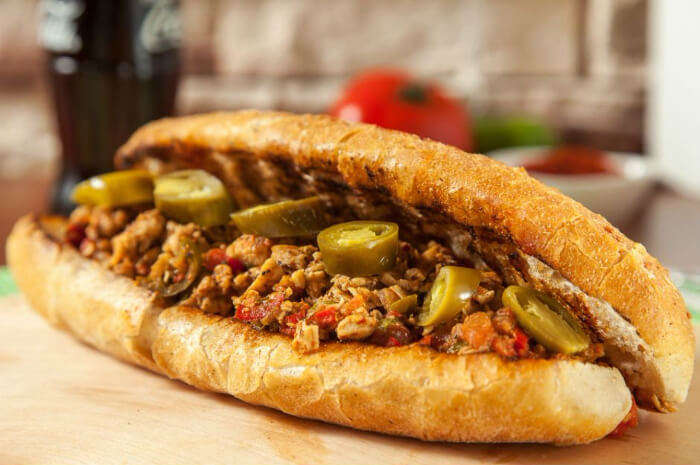This enticing, high-quality photograph captures a mouth-watering sub sandwich that looks perfect for sharing. The sub is made with seasoned ground beef and generously garnished with thick, cut-up jalapeno slices, adding a spicy kick. The bread is perfectly toasted to a beautiful golden brown on the outside, with a deliciously light char on the inside. The sandwich appears to be about six inches long, reminiscent of a homemade version of a sub you'd get from a shop like Subway, though this is clearly a custom creation.

The sandwich is resting on a rustic wooden cutting board, placed in a way that suggests it's ready to be enjoyed. In the background, a slightly blurred kitchen scene adds to the cozy, homemade feel of the image. The background also includes a nostalgic glass bottle of Coca-Cola, a whole tomato, and a bowl with an indiscernible ingredient, further enhancing the homey atmosphere.

This delectable ground beef and jalapeno sub is visually compelling and practically begs to be eaten, making it an ideal photo for Instagram.